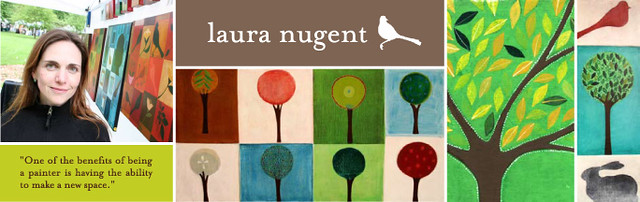This image is a wide, narrow rectangular banner, likely for a website or social media, featuring the artist Laura Nugent. The left-hand third of the banner displays a photograph of Laura, a young Caucasian woman with long brown hair, wearing a zipped-up black jacket. She is smiling slightly at the camera, sitting outdoors in front of a series of colorful paintings on display, with green grass and trees in the distant background. Beneath her photo, a green box with white or black text includes a quote from Laura: "One of the benefits of being a painter is having the ability to make a new space."

The center section of the banner has a light brown background with the name "Laura Nugent" in white print, accompanied by an illustration of a white bird in silhouette. Below this banner is a series of eight minimalistic paintings, each depicting trees with circular, lollipop-like tops in various color schemes. These paintings feature combinations like orange on brown, light green on dark green, red on white, and green on pink, each tree having a similar trunk but different colored backgrounds and foliage.

The right-hand section of the banner showcases additional artwork by Laura. First, there is a detailed painting of a tree with multicolored, uniformly shaped leaves and a dark brown trunk. Beside it, there are three more pieces: a tree with pink background and red bird, a tree on a blue background, and a stencil-like depiction of a gray bunny rabbit on a light background. These elements together highlight Laura's distinctive, minimalist artistic style and thematic focus on nature.